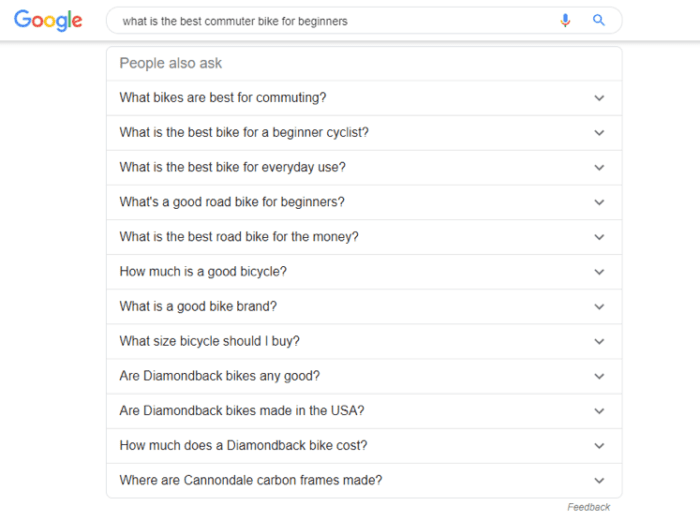The image depicts a Google search results page, likely viewed on a smartphone or computer. The Google logo is prominently displayed in the upper left corner, indicating the familiar search engine interface. The search query entered by the user is "What is the best commuter bike for beginners?" This query is flanked by a microphone icon and a blue search button on the right. Below the search bar is the "People also ask" section, consisting of a list of related questions with drop-down arrows to their right. 

The questions listed are:

1. What are the best bikes for commuting?
2. What is the best bike for a beginner cyclist?
3. What is the best bike for everyday use?
4. What's a good road bike for beginners?
5. What is the best road bike for the money?
6. How much is a good bicycle?
7. What is a good bike brand?
8. What size bicycle should I buy?
9. Are Diamondback bikes any good?
10. Are Diamondback bikes made in the USA?
11. How much does a Diamondback bike cost?
12. Where are Cannondale carbon frames made?

The text of these questions is left-justified. At the very bottom right of this section, underneath all the drop-down arrows, there is a small, light gray text link labeled "Feedback." The background of the page is solid white, making the text and elements stand out clearly.